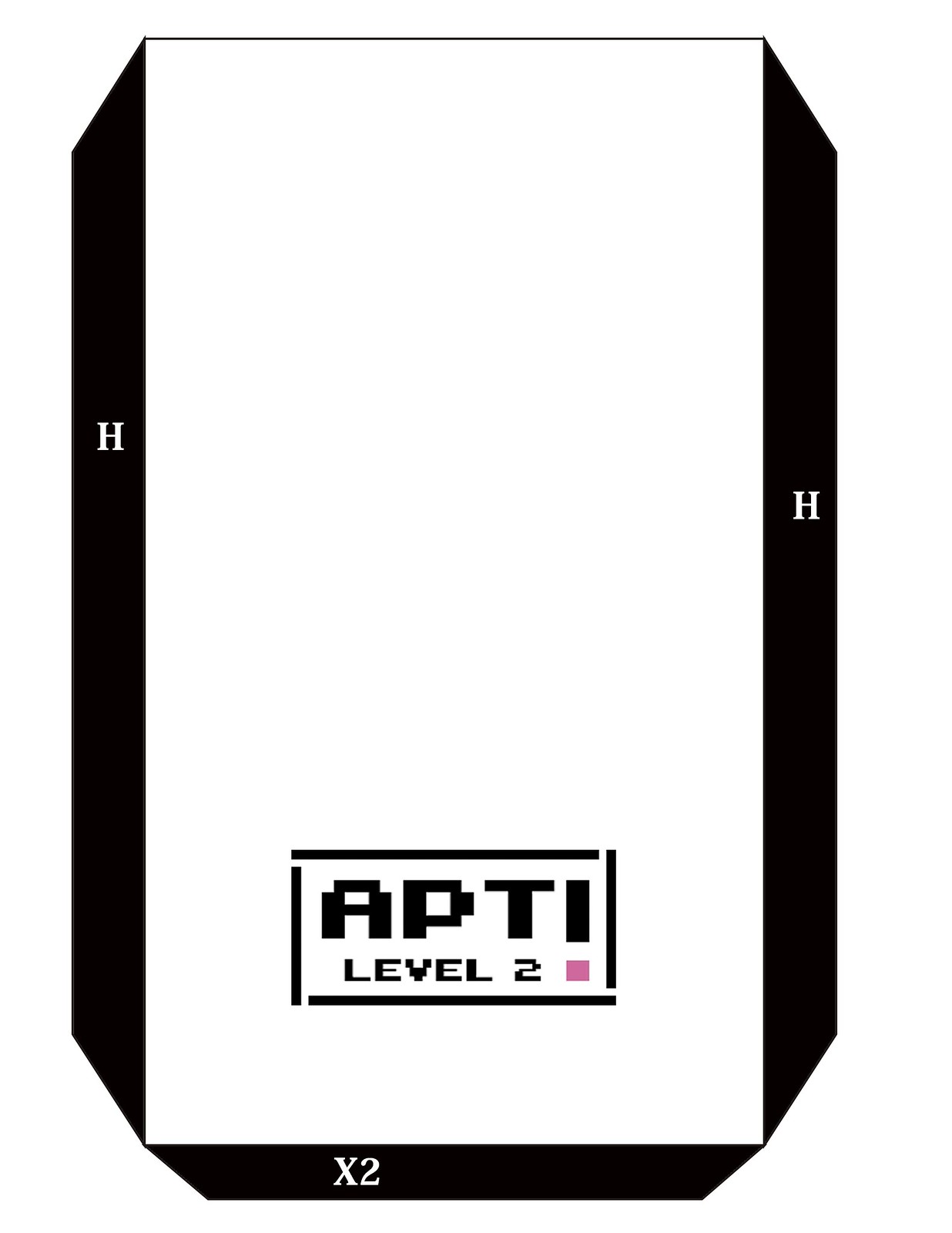This is a very intriguing vintage-style black and white image, possibly from a video game or a manual. Predominantly white, it features a large vertical rectangle in the center. On each side of this rectangle, there are black tabs: one on the left with a white letter 'H', and one on the right with another white 'H'. At the bottom of the central rectangle, there's a black tab marked with 'X2' in white. Inside the large rectangle, we see the letters 'A', 'P', 'T', followed by an exclamation mark (or possibly an 'I'), written in a pixelated font reminiscent of early video games. Below this text, it says 'level 2', also in pixelated style. There is a small, distinct pink box situated next to the number '2'. The image exudes a nostalgic feel due to its pixelated and vintage appearance, yet its purpose remains ambiguous.